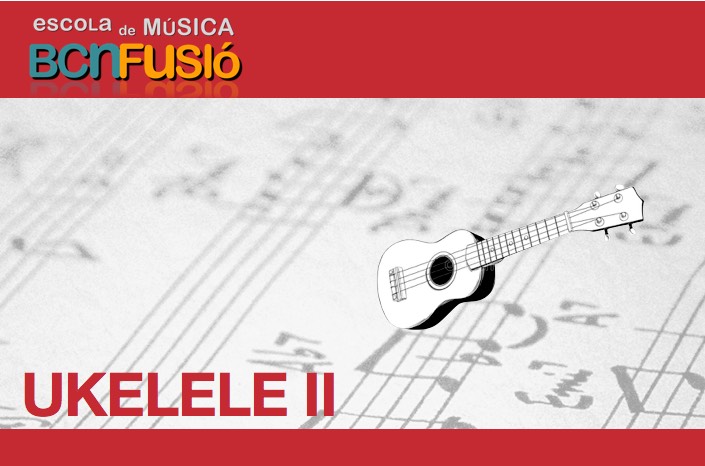The image appears to be a digitally designed poster advertising a music class. It is dominated by a background of sheet music, which looks realistic, displaying a music staff with notes written in a foreign language. At the top of the poster is a red banner with the text "Escola de Música BCN Fusió". Another red border runs across the bottom of the image. Just above this bottom banner, "Ukulele 2" is prominently written in bold, red letters. On the right side of the sheet music, there is a detailed black and white illustration of a ukulele, distinguishable by its four strings and central sound hole. The overall composition suggests a blend of photographic elements and hand-drawn art, creating a visually engaging advertisement for a music class or program.